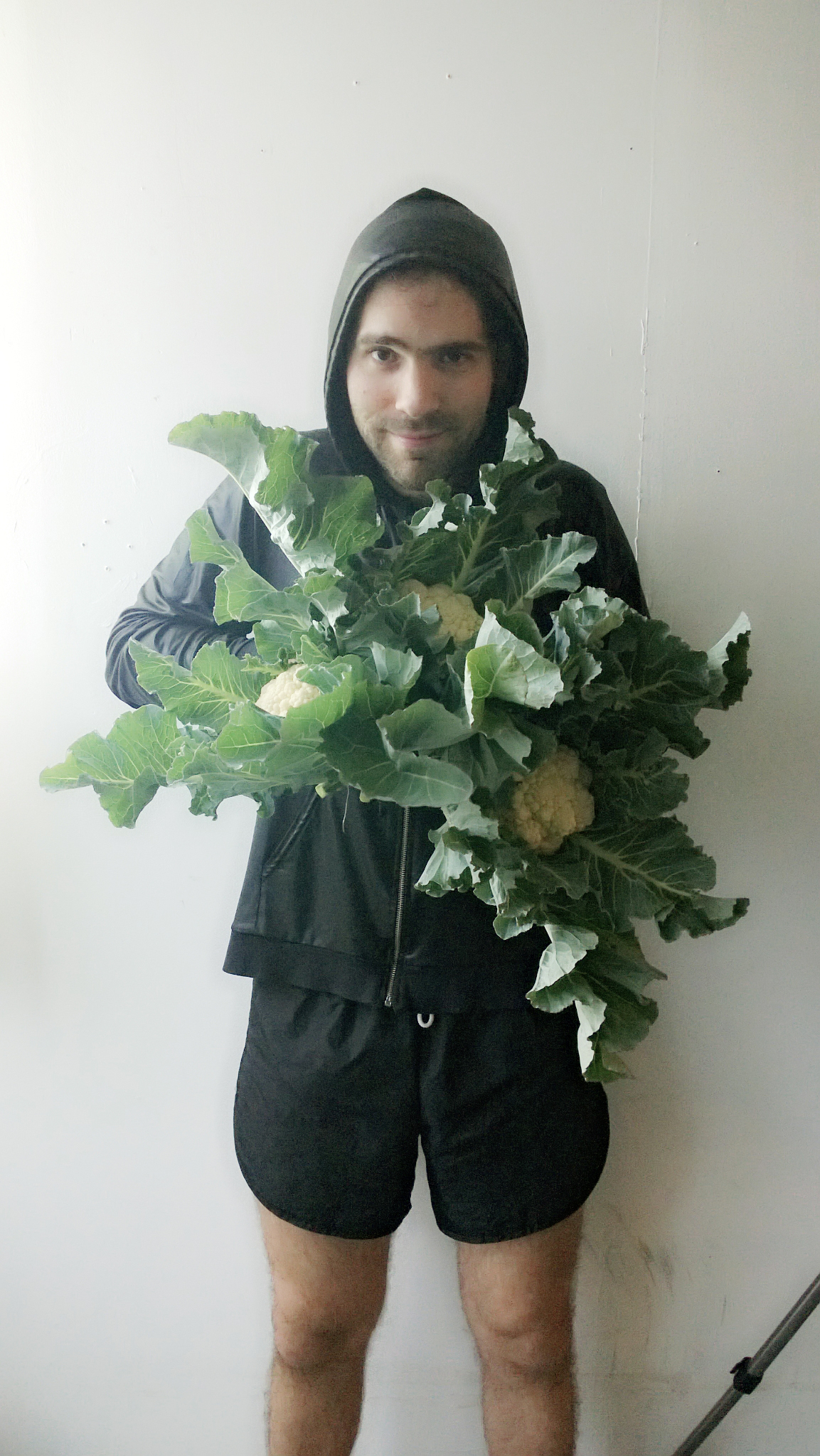A digital photograph captures a vertical image of a man, who appears to be in his 30s, standing against a predominantly white background with some variation in brightness due to lighting. He occupies almost the entire height and width of the photo. The man, who has medium-toned skin, defined by his visible 5 o'clock shadow with brown stubble on his chin and above his lip, is dressed in a black hoodie with the hood up and black shorts that extend just above his knees. His look is accented by his expressive eyebrows, with his left eyebrow raised. He gazes directly into the camera. In his arms, he holds large, leafy vegetables that resemble cauliflowers, characterized by crumbled green leaves and central reddish or whitish cauliflower heads. Additionally, a black metal rod or tripod leg can be seen diagonally across the lower right-hand corner of the photograph, holding a small black square piece in its midsection.